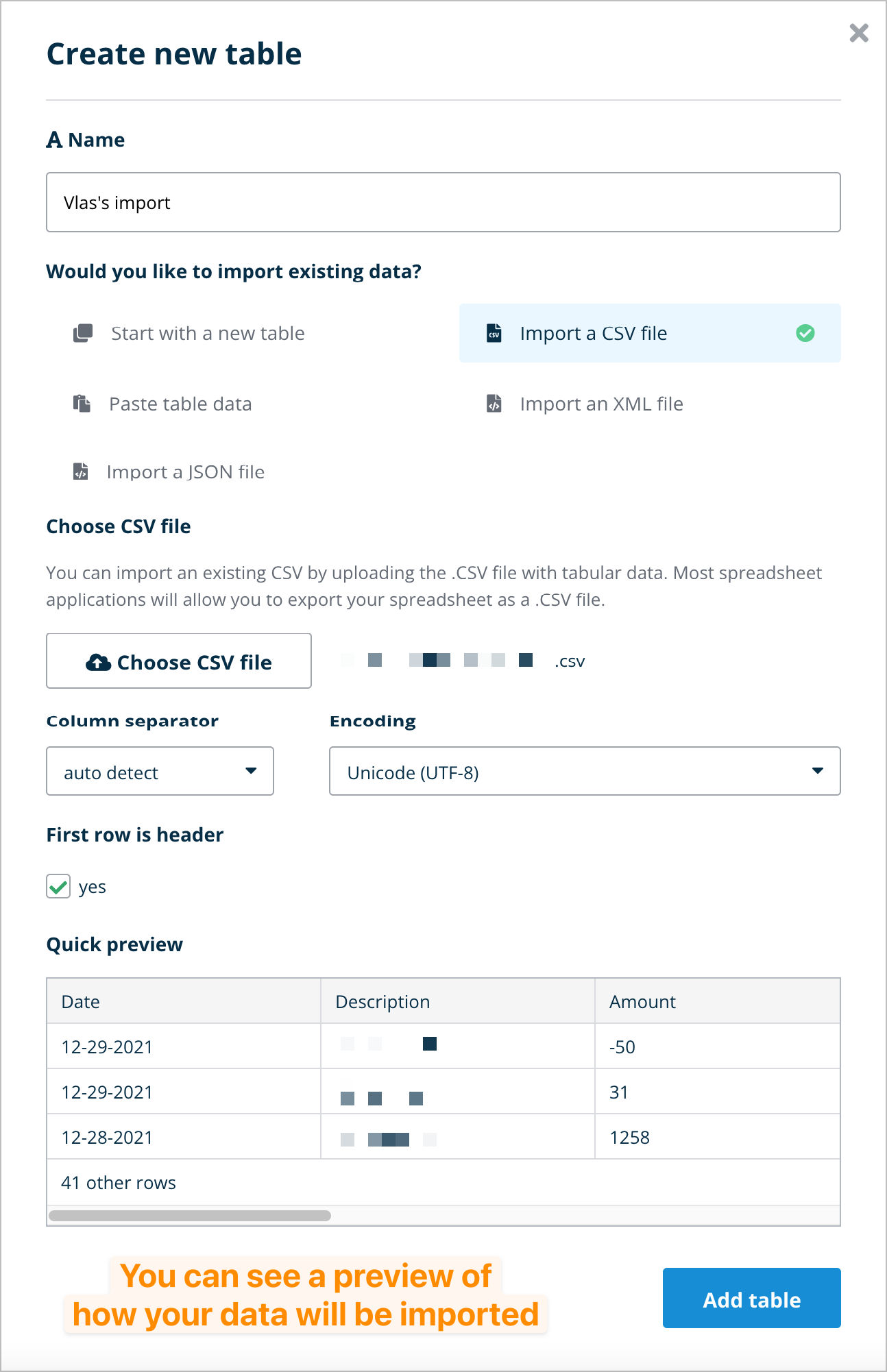The image displays a user interface with a layout approximately twice as tall as it is wide, framed by a black border. At the top left corner, bold black text reads "Create New Table," indicating that the image shows an interface likely from an application designed for table creation or data management. A gray 'X' is present in the upper right corner, suggesting a close or exit button.

Below the title, there is a gray horizontal bar followed by the text "Unname" in black, which appears to be a placeholder for entering a table name. A field beneath "Unname" is filled with the text "V-L-A-S's import."

Further down, bold black text asks, "Would you like to import existing data?" This question is followed by several clickable options arrayed in two columns. The left column lists:
1. "Start with a new table."
2. "Paste Table Data."
3. "Import a JSON file."

The right column contains:
1. "Import a CSV file."
2. "Import an XML file."

Each option is accompanied by an icon on its left and light gray text describing the action. "Import a CSV file" is selected, as indicated by a green check mark and a light blue outline around this option.

Below these choices, more bold black text reads "Choose CSV file." This is followed by a paragraph providing details on the process, and an upload button displaying a cloud icon. The button text also reads "Choose CSV file," inviting the user to select a file for upload.